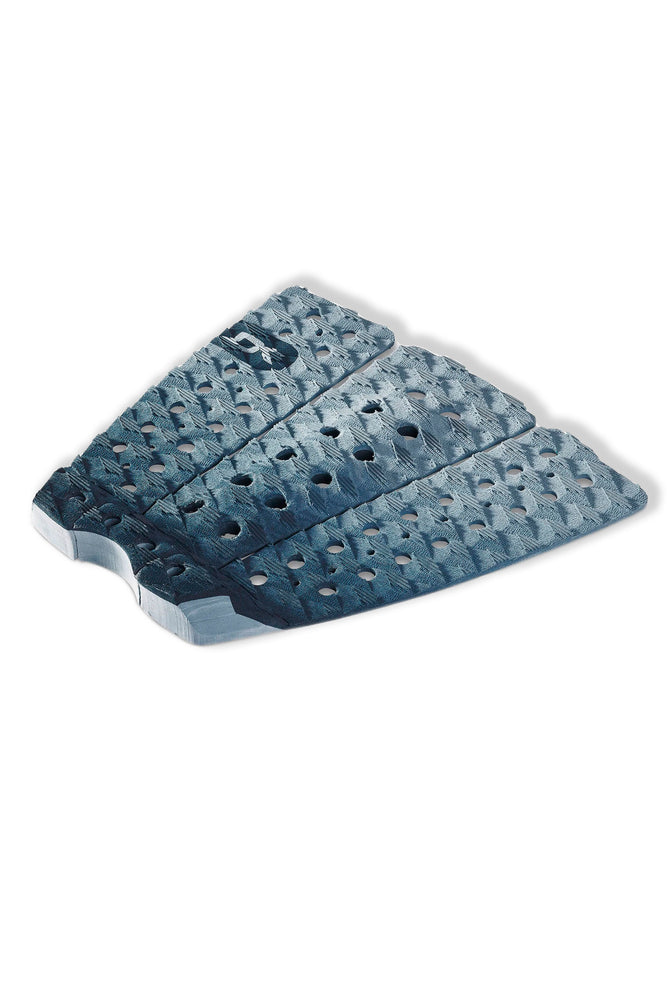The image depicts a product consisting of three rectangular, interconnected sections resembling long, thin swimming flippers without the flared ends. These sections, which taper slightly from left to right, are a light bluish-gray color and feature rows of circular holes. The outer sections have two rows of nine large holes each, with smaller holes interspersed in between. The central section, slightly wider than the outer ones, has two rows of six large holes. Each of these rows is aligned in a neat row with additional smaller holes in the spaces between them. The sections are all oriented towards the top right. Notably, there is a logo in the upper left corner that resembles the letters "D" and possibly "L" or "K". The detailed design and specific features suggest this could be a type of tile or flooring material, possibly intended for use in a bathroom or other tiled area.